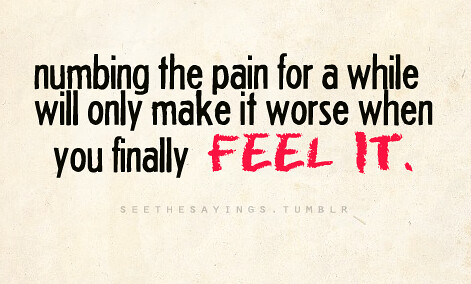The image is a Tumblr quote post featuring a vintage-style, light beige background that gives off a slightly yellowish tone. The focal point of the image is the quotation: "numbing the pain for a while will only make it worse when you finally feel it." The majority of the text is in black, lowercase, and uses a simple sans-serif font. However, the last two words, "feel it," are in bold, all-capitalized red letters, rendered in a distinctive, handwritten typeface that captures immediate attention. Below the quote, in grayed-out, all-capital letters, it reads "see the sayings dot tumblr," indicating the source of the post. The text occupies about two-thirds of the image, making the message prominently visible.